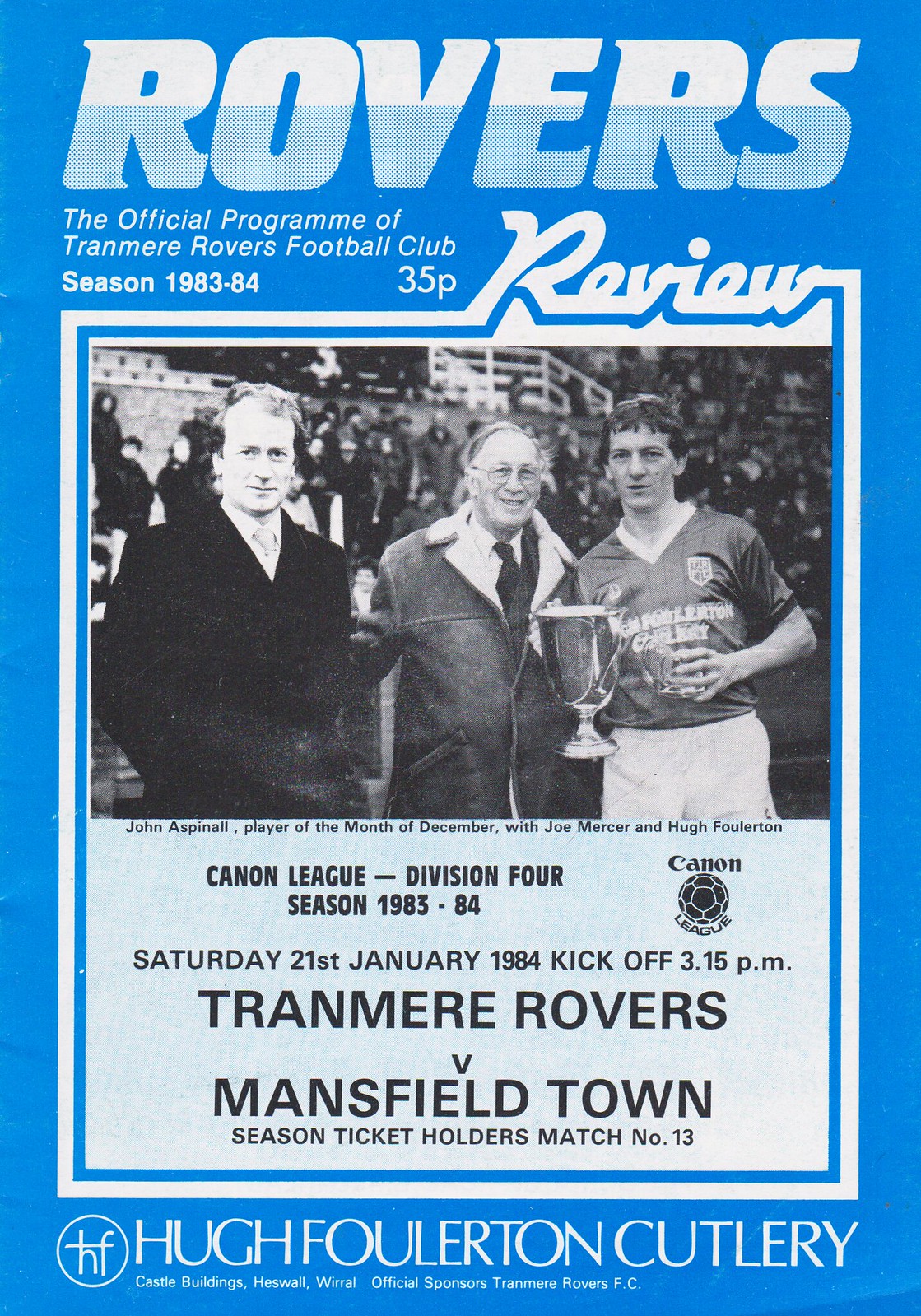This vintage poster from the 1983-84 season of the Tranmere Rovers Football Club features a light bluish background with prominent white letters at the top spelling "ROVERS." Below that in large letters, it declares the "Official Programme" of the club, priced at 35P. To the right, in a white outline, the word "REVIEW" stands out. 

At the center, a black-and-white photograph captures three individuals: on the left, a man in a suit with a white collared shirt and tie; in the center, an older gentleman wearing glasses and a greyish overcoat with a white fur trim; and on the right, a football player holding a trophy in his right hand and possibly a glass in his left hand, dressed in a football jersey and white shorts. The caption identifies the individuals as John Aspinall, player of the month for December, alongside Joe Mercer and Hugh Fullerton.

Below the photo, black writing announces details for an upcoming match: "CANNON LEAGUE - DIVISION 4, Season 1983-84," with "CANNON" accompanied by a soccer ball symbol. It continues with "SATURDAY 21ST JANUARY 1984, KICKOFF 3.15 PM," for the match "TRANMERE ROVERS VERSUS MANSFIELD TOWN." Further down, it notes "Season ticket holders match number 13." At the very bottom, sponsors are acknowledged with the text: "Hugh Fullerton Cutlery," and some smaller, less distinct lettering.